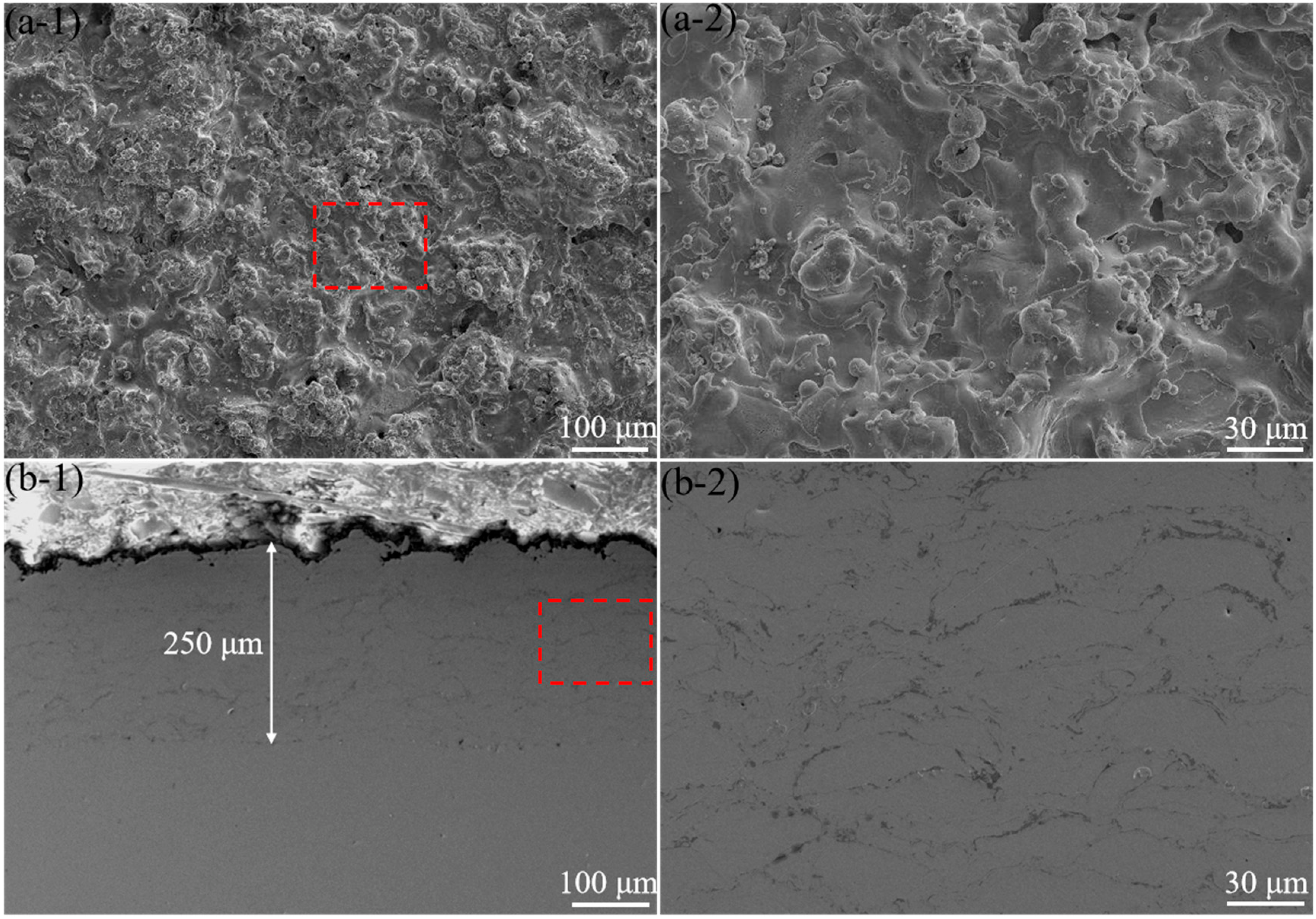The image comprises four satellite photos arranged in a square grid with two on top and two on the bottom. Each photo is labeled distinctly: the top-left as A1, the bottom-left as B1, the top-right as A2, and the bottom-right as B2.

In each image on the left side (A1 and B1), a red dashed square highlights a specific area. Both A1 and B1 have labels indicating "100 UM" in white text. Conversely, the right side images (A2 and B2) lack the red dashed squares but are labeled "30 UM" in white text. Additionally, B1 is marked with a white arrow pointing to "250 UM”.

The visual content is intricate and somewhat abstract: 
- A1 and A2 exhibit a meshwork of gray and white squiggly lines, challenging to interpret.
- B1 resembles ocean waves lapping at a shoreline, enhanced by the "250 UM" annotation.
- B2 evokes the appearance of mud with discernible circular formations.

This detailed caption contextualizes the technical aspects and visual impressions of the satellite images for a comprehensive understanding.